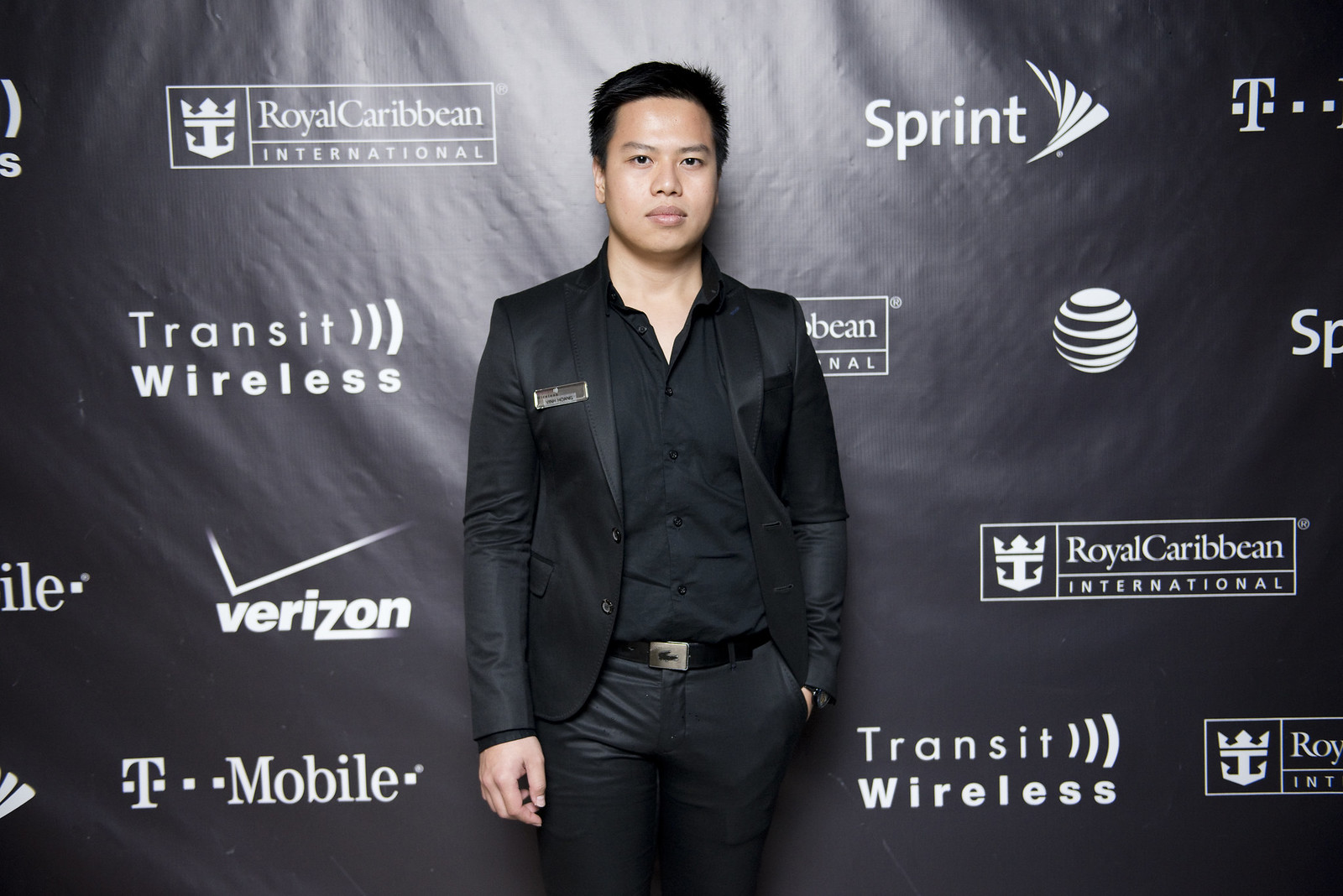The image is a color landscape photograph featuring a young Asian man in his late 20s, standing in front of a black ad wall at a premiere event. The wall behind him showcases white logos of various sponsors, including Royal Caribbean International, Transit Wireless, Verizon, T-Mobile, Sprint, and AT&T, with some repeating. The man is centrally positioned, facing the camera with a neutral expression. He is dressed in an entirely black ensemble, including a black suit jacket, a black button-up shirt, black pants, and a black belt with a silver buckle. A name tag is affixed to his right lapel. His left hand is in his pocket while his right hand hangs by his side. The photograph is captured in a realistic, representational style, highlighting the details of both the subject and the backdrop.